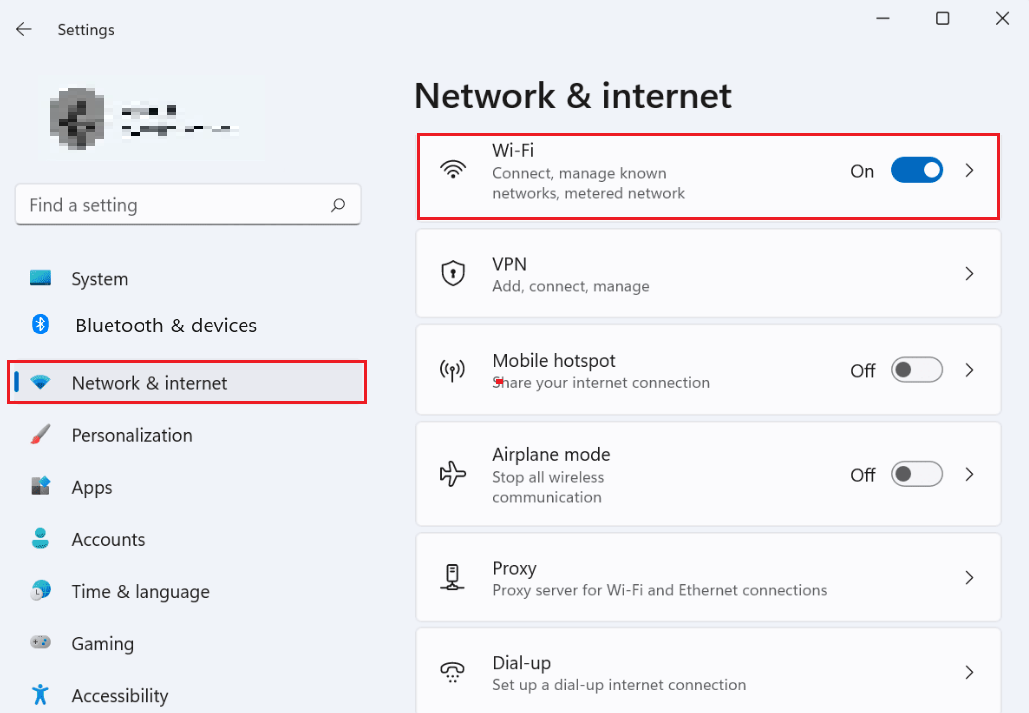A detailed caption for an image of a settings page in the Windows operating system:

This image features a screenshot of the "Network & Internet" settings page in Windows. The interface has a light blue-gray background with black text. The page has a rectangular shape. 

On the right side of the image, there are six rectangular boxes aligned vertically, each with a white background displaying various network settings. The first box, highlighted with a red outline, is labeled "WiFi" and includes a toggle switch currently turned on. The subsequent boxes are labeled "VPN," "Mobile Hotspot," "Airplane Mode," "Proxy," and "Dial-Up."

In the top left corner of the screen, the word "Settings" is displayed next to a left-facing arrow, suggesting a navigation option to return to the previous page. At the center top of the screen, in bold text, is the title "Network & Internet," indicating the current section. 

Running vertically down the left side of the screen is a navigation menu with multiple options. It begins with a search bar labeled "Find a setting." Below the search bar, various settings categories are listed: "System," "Bluetooth & devices," and "Network & internet," which is outlined in red to show that it is the currently selected category. Following these are "Personalization," "Apps," "Accounts," "Time & language," "Gaming," and "Accessibility."

This detailed layout shows ease of navigating through the diverse network and connectivity settings available on a Windows PC.